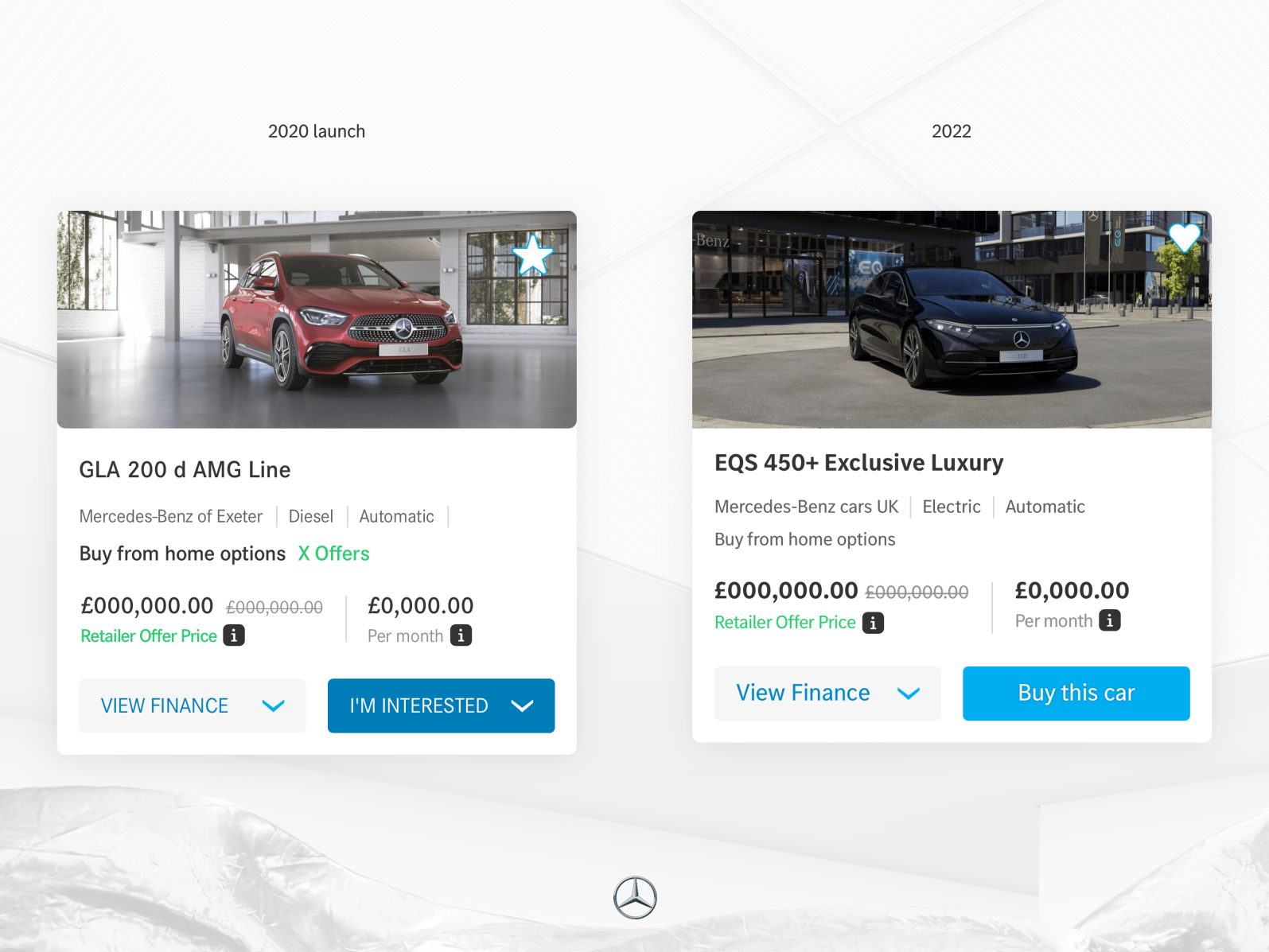A screenshot from a website featuring a gray background with a faint graphic image resembling folded fabric. The web page displays two listings side-by-side, labeled in black font at the top. The listing on the left is titled "2020 Launch" and the one on the right is labeled "2022."

The "2020 Launch" listing showcases a red Mercedes sedan parked in a showroom. The details below the image specify "GLA 200d AMG Line, Mercedes-Benz of Exeter, Diesel, Automatic." It also offers "Buy from home options," but the price is erroneously displayed as "$000,000.00," indicating a mistake. Additional buttons are available for viewing financing or expressing interest.

The "2022" listing features a black Mercedes sedan with the model "EQS 450+ Exclusive Luxury" described below the image.